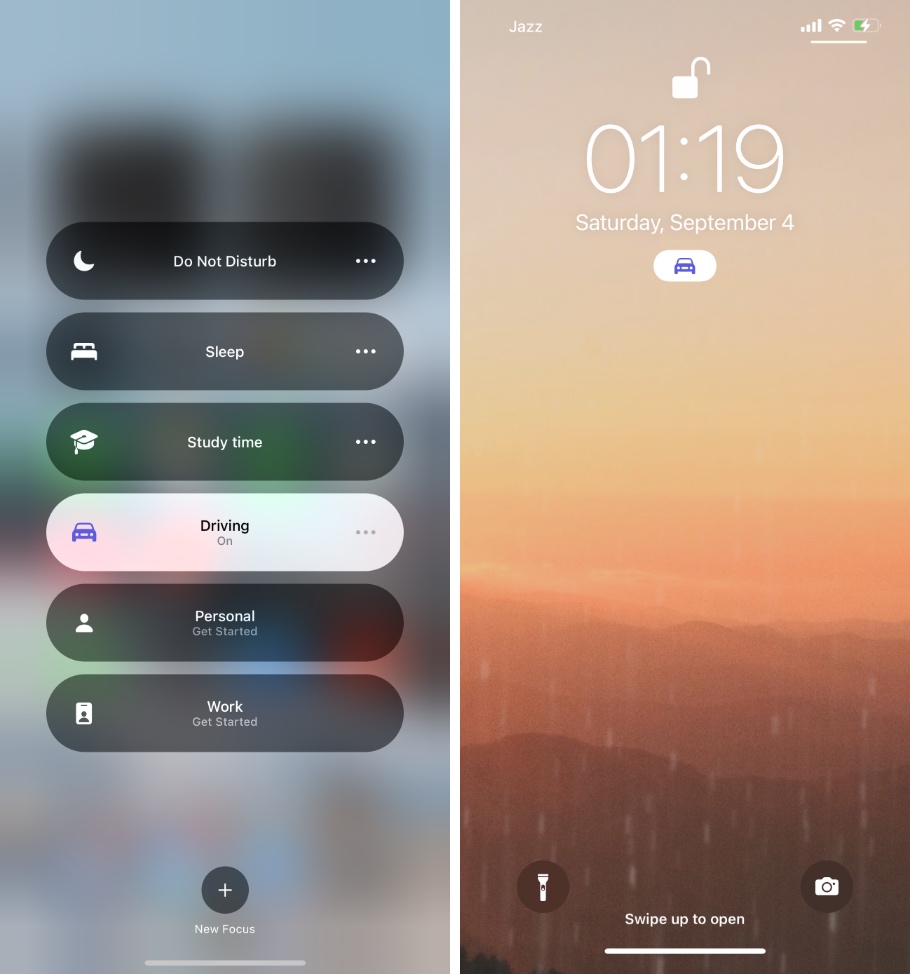The image is divided into two panels. On the left panel, the background is creatively blurred, transitioning from blue at the top to gray at the bottom, with hints of rainbow colors. Six elongated ovals with soft edges are prominently displayed. The first oval features a moon icon alongside the text "Do Not Disturb." Following this, the second oval displays a bed symbol with the word "Sleep." The third oval includes a graduation cap icon and the label "Study Time." 

Moving on, there's a white-background oval with a purple car icon, indicating "Driving," which is currently turned on. The fifth oval returns to a gray background, labeled "Personal." The sixth oval features a motivational message, "Work, Get Started." At the bottom, there is a gray circle with a plus sign and the text "New Focus" in white print.

The right panel shows a computer screen interface. At the top, the word "Jazz" is displayed alongside battery, cell signal, and WiFi indicators. Centrally, there is an unlocked padlock icon, followed by the date and time: "00:19, Saturday, September 4th." Below this, an oval with a purple car icon is visible. The background color shifts from peach at the top to dark red at the bottom. In the center, icons for a flashlight and a camera are shown, accompanied by the instruction "Swipe up to open."